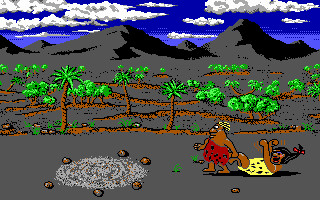The image is a detailed digital screenshot from an old video game, reminiscent of classic floppy disk titles possibly like "Caveman Olympics". It features a blue sky studded with white clouds and a backdrop of shadowed, gray mountains devoid of snow. The terrain beneath is completely gray, adding a stark contrast to the vibrant elements depicted. In the scene, various green-leaved trees, including palm trees and smaller shrubs, dot the landscape. 

Central to the image is a caveman with dark skin, clad in a red animal print outfit adorned with black dots that drapes over one shoulder. He has blonde hair and is facing left. This caveman is seen dragging a cavewoman by the leg. She is on her back, her head turned to the right, smiling, with her hands raised in a gesture devoid of distinguishable fingers. She sports long black hair tied with a red bow and wears a yellow animal print dress. The caveman appears to be moving towards a circular, stone-bordered pit that resembles a swirling sand vortex. The image's pixel art style suggests it was created for a handheld device or an early computer game, with tiny, pixelated graphics that almost resemble a GIF.